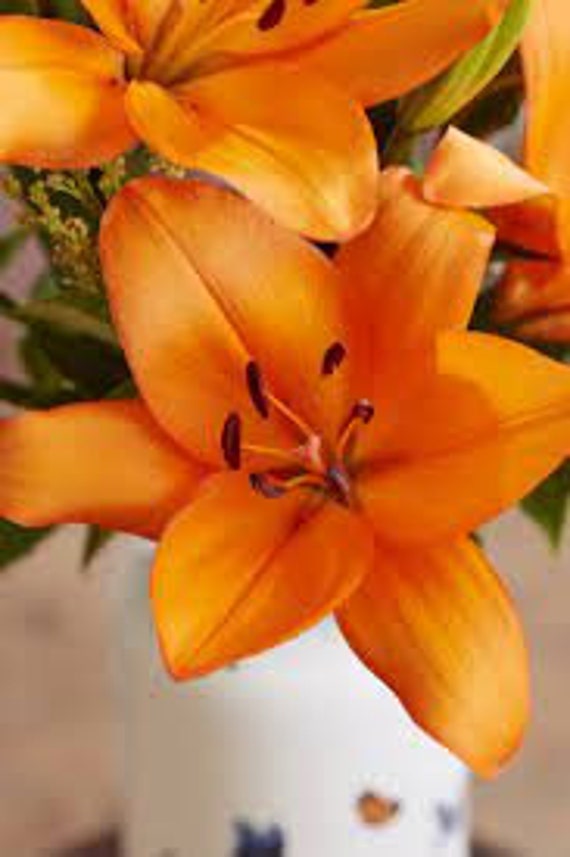This close-up photograph captures a vibrant display of flowers, likely from the lily family, characterized by their bright yellowish-orange hue. Each flower prominently shows two sets of petals arranged in groups of three, forming an elegant overlay. The central part of each bloom exhibits six conspicuous stamens. The image, though blurry and pixelated, reveals the flowers sprouting from a shiny, white enamel or metal pot adorned with small, colorful figures or patterns. Behind this, green foliage is visible, set against a dimly lit room, devoid of identifiable features. Despite the quality of the photograph being poor, the intricate details of the flowers and their container stand out clearly.